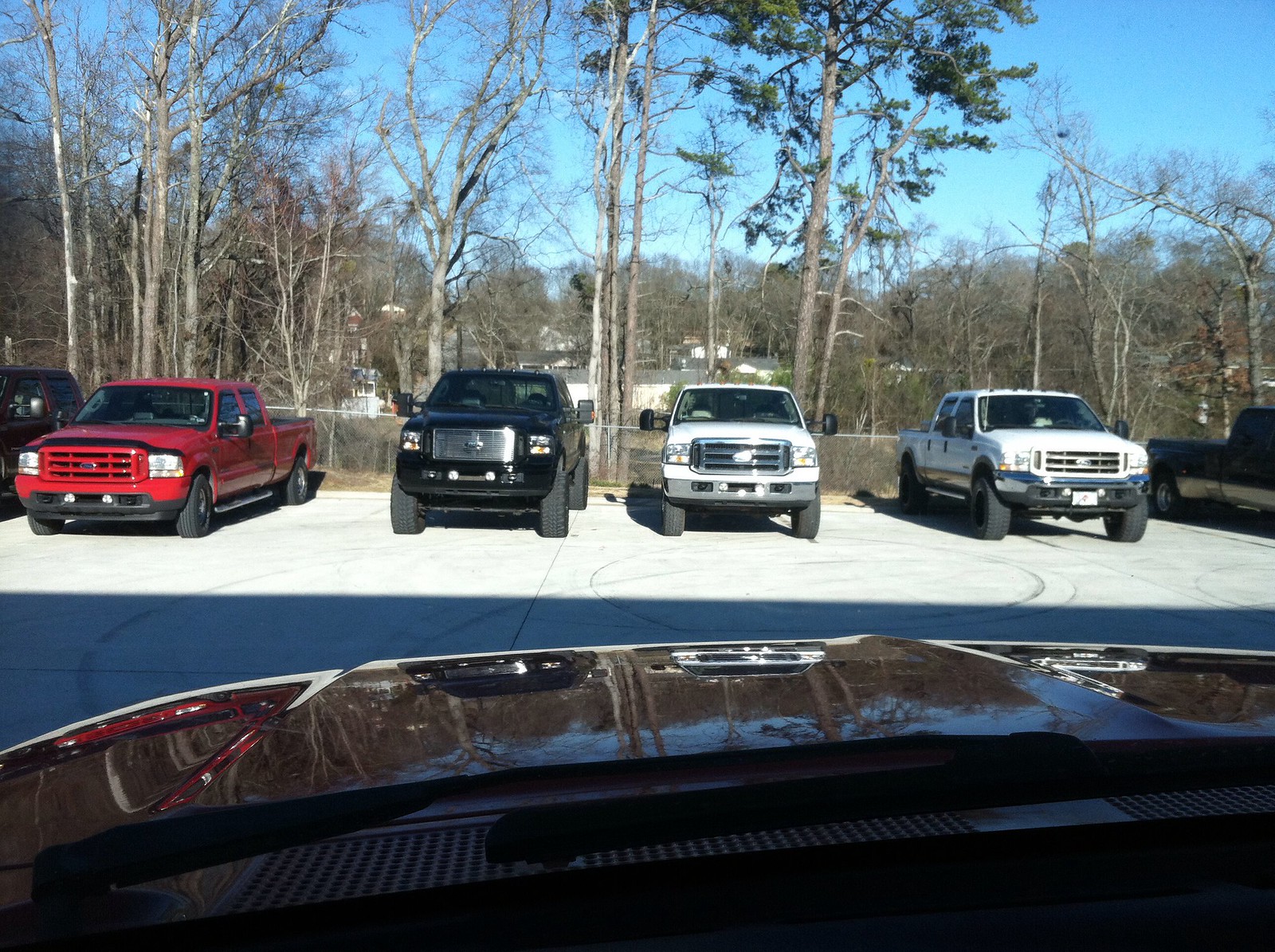This photo captures the view from inside a vehicle, likely taken through the windshield of a truck. It reveals a parking lot scene with several Ford pickup trucks arranged in a row. Starting from the left, you can barely see the edge of a brown truck, followed by a prominently visible red truck, a black truck, two white trucks, and a glimpse of a dark truck at the far right. These trucks, most of which are extended cab models with larger back seats and tail beds, are situated on blue and white pavement, indicating some variation in the ground surface. Three of the trucks are jacked up higher than the lower-sitting red truck. In the background, there are tall pine trees mixed with mostly bare trees, with one tree near the center-right still bearing leaves. The sky transitions from a darker blue at the top to a lighter hue near the horizon. Additionally, residential houses can be seen beyond the treeline, suggesting the parking lot is adjacent to a residential area.